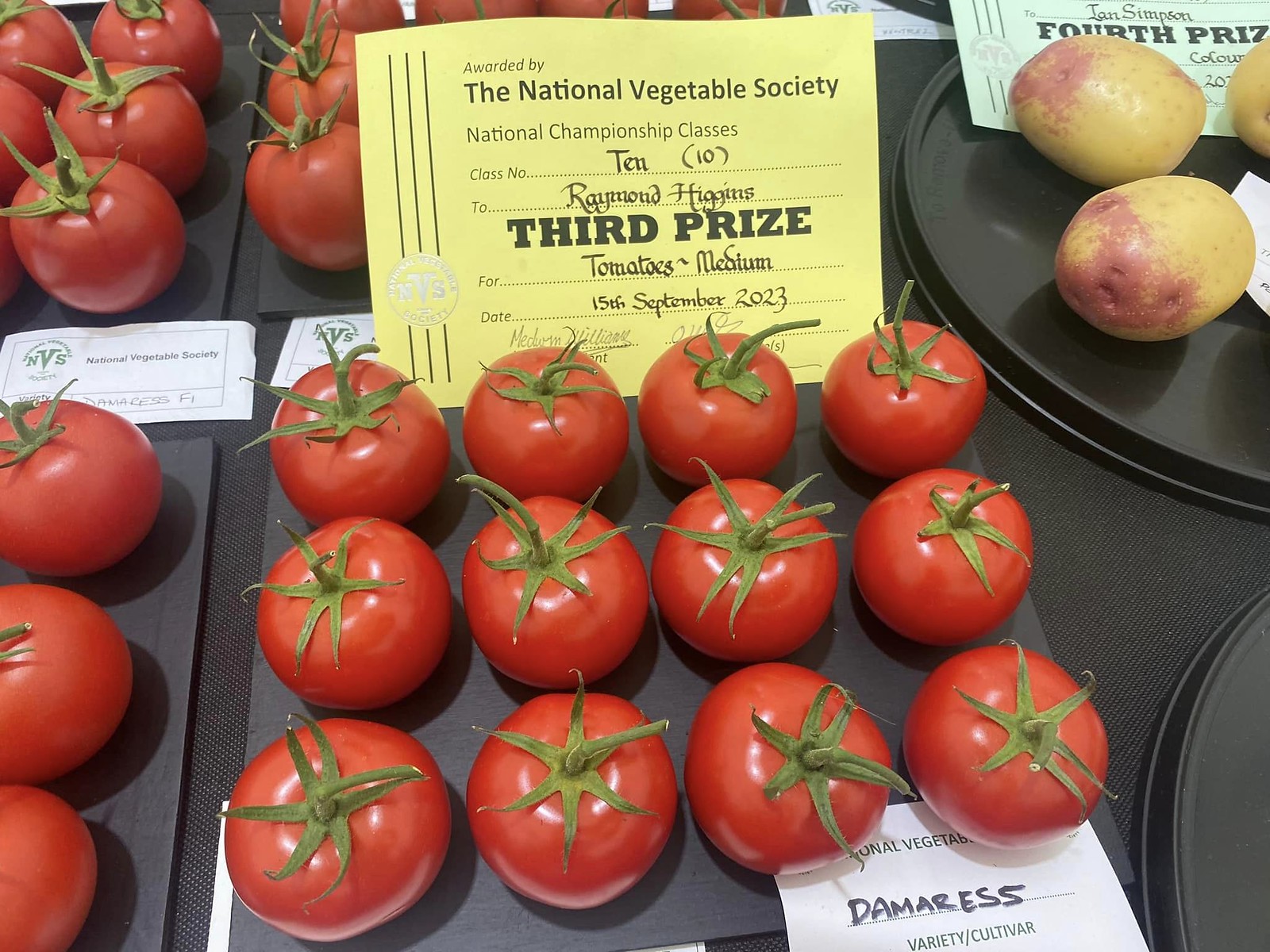This photo captures the National Vegetable Society's contest, centered on an array of award-winning produce. Dominating the scene in the middle is a tray holding twelve vibrant red tomatoes with lush green stems. Above this tray sits a yellow certificate that reads, "Presented by the National Vegetable Society, National Championship Classes, 10 Raymond Haynes, Third Prize, Tomatoes Medium, September 15th, 2023." Surrounding this central display are more collections of similarly striking tomatoes. In the upper right corner, a partially visible fourth-place certificate indicates recognition for yellow vegetables, likely squash or potatoes, awarded to Jan Simpson. The overall image brims with carefully arranged, prize-winning vegetables, showcasing the proud achievements of the contestants.